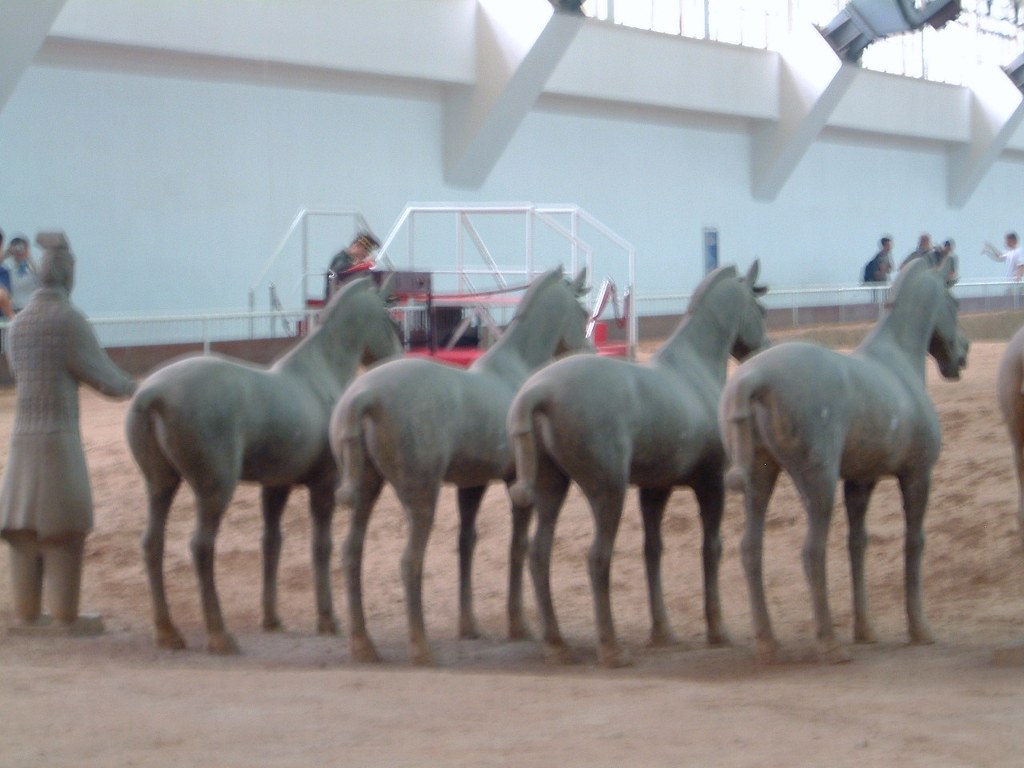This outdoor photograph captures a scene of what appears to be a display or exhibition featuring statues of a terracotta warrior and four terracotta horses, set against a sandy foreground that resembles a rodeo or corral area. The statues are arranged with the warrior in a long coat and pants standing behind the horses, which are made of a stone-like material. Notably, one of the horses has a broken tail. The background reveals a white tall wall stretching from east to west, interspersed with windows allowing sunlight to penetrate the scene, creating a slightly blurred effect on the people gathered on a ramp that runs parallel to the wall. A red truck is also positioned in the foreground. The photograph, though a bit blurry and of lower quality, vividly captures the intricate details of the statues and the ambient setting, suggesting it was likely taken for personal enjoyment to document the experience of seeing these remarkable displays.